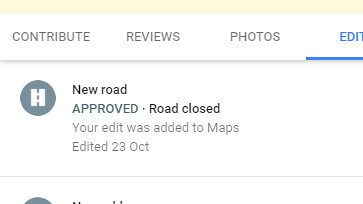Detailed Caption:
The image appears to be a cropped screenshot, likely taken on an iPhone, showing a small section of a user interface, possibly from a mapping or navigation app. At the top of the screenshot, there's a long, slender bar with a peach background color. Directly beneath this bar, in gray, uppercase letters, the words "CONTRIBUTE REFUSE PHOTO" are clearly displayed, each separated by spaces. Below this line, in a lighter blue font, the word "EDIT" stands out, followed by a gray horizontal line which turns light blue directly under the word "EDIT."

The next section of the image displays a circular icon featuring a two-lane road with dotted lines in the center. To the right of this icon, the text "NEW ROAD" is written in black. Adjacent to it in capital letters are the words "APPROVED. ROAD CLOSED." Additional text reads "Your edit was added to maps, edited 23 October," conveying that a user contribution was integrated into a map on that date. Immediately below this text is another slender line, followed by the beginning of an additional line that trails off into indistinguishable dots, suggesting the continuation of information that is not fully visible in the screenshot.